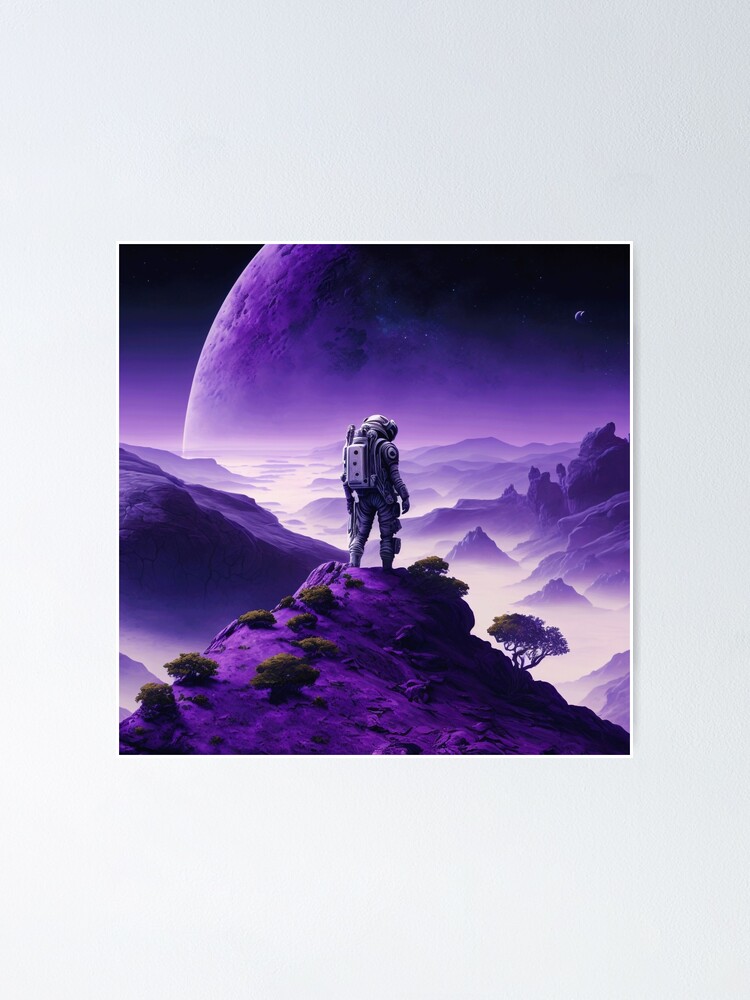The image is a sci-fi themed artwork that presents a portrait-style landscape with an ethereal, slightly surrealistic atmosphere. At the center of the image, a solitary figure in a modern astronaut suit stands atop a cliff, facing away from the viewer towards a two o'clock position. The figure’s position and attire suggest a sense of exploration and solitude. 

The dominant color scheme is composed of various shades of purple, creating a mystical and otherworldly ambience. The ground underfoot is a purple-tinted terrain with patches of sparse green vegetation. Stretching into the distance, the landscape features more purple hills and mountains that fade into the horizon.

In the sky, occupying much of the background, is a massive celestial body that appears to intersect dramatically with the horizon, almost as if it is about to collide with the planet the astronaut is on. This massive planet, or moon, is barren and uninhabited, with a surface that provides a stark, contrasting backdrop to the vivid foreground. Scattered stars dot the sky, heightening the alien environment, though the overall scenery remains bleak and desolate.

No facial features or other specific identifying characteristics of the astronaut can be discerned, adding to the mysterious quality of the image. The scene is enveloped in a hazy, dream-like quality, suggesting that it may be an imaginative creation rather than a depiction of a real place, possibly crafted by an artist with a passion for science fiction.